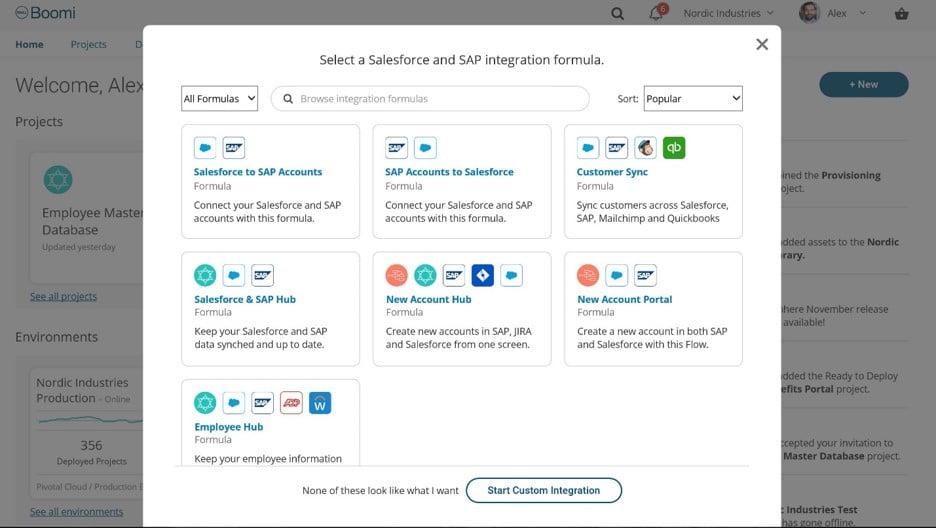The image features a variety of elements and symbols related to business software integration, prominently showcasing both icons and descriptive text. In the top left corner, "Boomi" is displayed, while the top right corner features a magnifying glass icon, a bell icon, and the text "Six" next to "Nordic Industries."

Nearby, there are multiple references to "Alex" and "Home," as well as dedicated sections for "Projects," "Alex," "Alexa," and "Ubuntu." Various statuses such as "New," "Employee," "Master Database," "Updated," and "Today" are mentioned, along with specific project names like "CL Projects," "Environment," and "Production." The number "256" is associated with "Deployed Projects."

Additionally, the image contains various instructional texts on integrating Salesforce and SAP systems. These include selecting and managing integration formulas like the "Salesforce to SAP accounts formula," the "SAP accounts to Salesforce formula," and the "Customer sync formula," which syncs customer data across Salesforce, SAP, MailChimp, and QuickBooks. There’s also a "Salesforce and SAP Hub formula" for keeping data consistent and "New account Hub formula" that simplifies creating new accounts across SAP, Jira, and Salesforce.

The "Employee Hub formula" is designed to manage employee information. Amidst the detailed instructions, the text reflects the user's indecisiveness: "None of these look like what I want."

Finally, the image includes an array of icons representing various software tools, such as the recognizable MailChimp logo featuring a monkey wearing a hat.